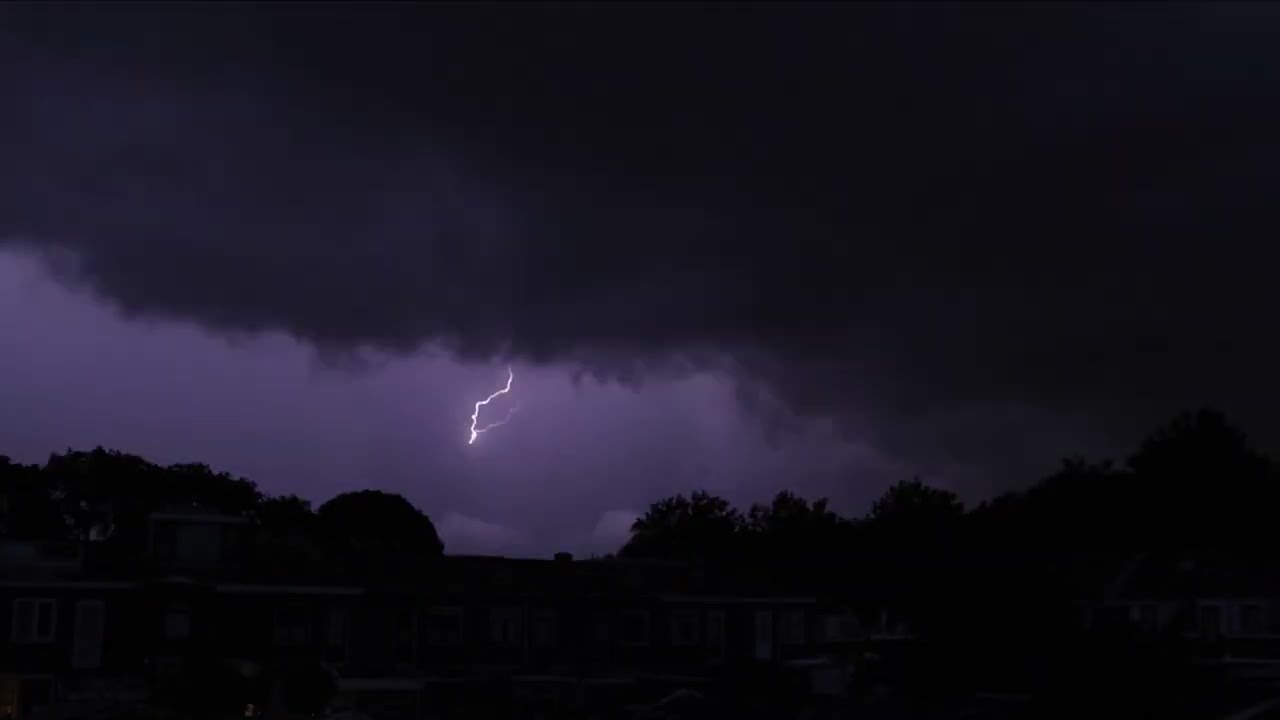In this image captured outdoors in the middle of the night, a dramatic thunderstorm dominates the scene. The sky is filled with dark, menacing clouds that appear in deep shades of gray and black, with a striking purple hue illuminating the background. Centered in the image is a vivid bolt of lightning zigzagging through the sky, illuminating the clouds and creating a stark contrast against the surrounding darkness. This primary streak of lightning does not reach the ground; it extends halfway from the clouds, accompanied by a fainter, trailing return streak. Below, the landscape features ominous silhouettes of trees that enclose the area, as well as outlines of multiple houses with faintly visible windows and doors. The scene’s foreground reveals a flat meadow under the lightning bolt, with additional trees to the right. The overall atmosphere conveys the intensity and turbulence of a night-time thunderstorm, with natural elements overshadowing human-made structures.